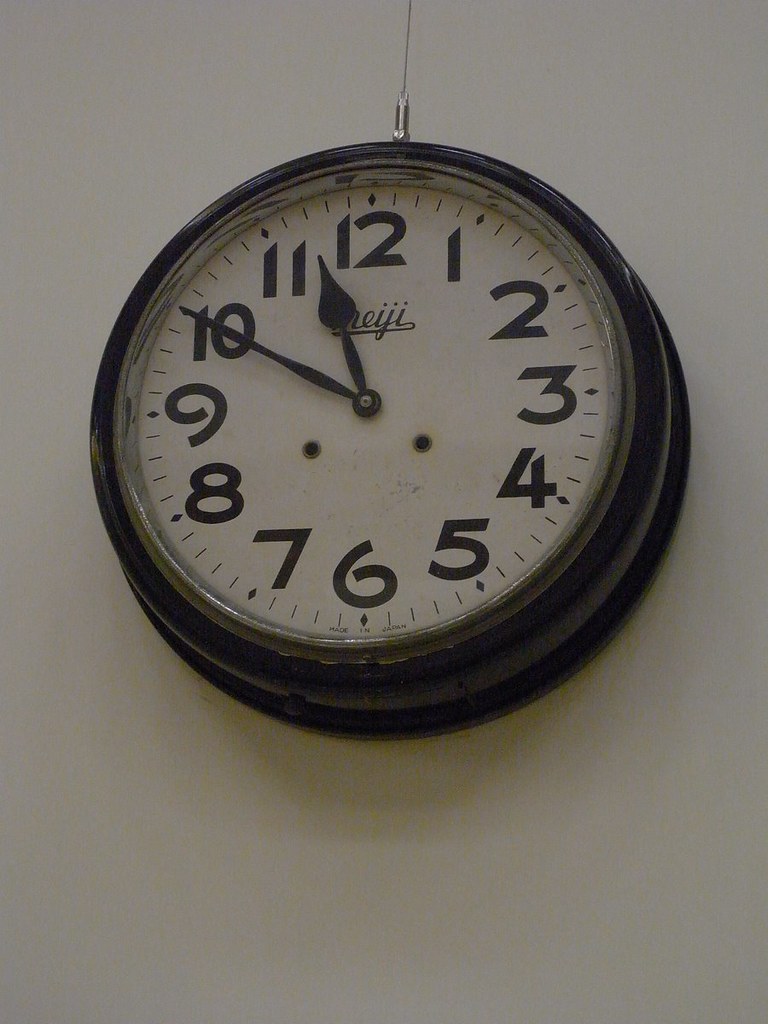This detailed image captures an older, well-worn analog clock with a distinctively artistic appearance. The clock is circular with a black outer frame and has a silver metal ring inside. The face of the clock is white, covered with glass, and features black Arabic numerals. Notably, there are two black hands: a small hand just past the 11 and a large hand on the 10, indicating the time is 11:50. The clock face includes two small holes for winding via a key. Above the center, beneath the number 12, a label in cursive reads "Meiji," suggesting the manufacturer's brand, with a faintly underlined text. The entire clock is suspended on the off-white wall by a silver metal wire or fastener, which adds to its vintage yet functional aesthetic.